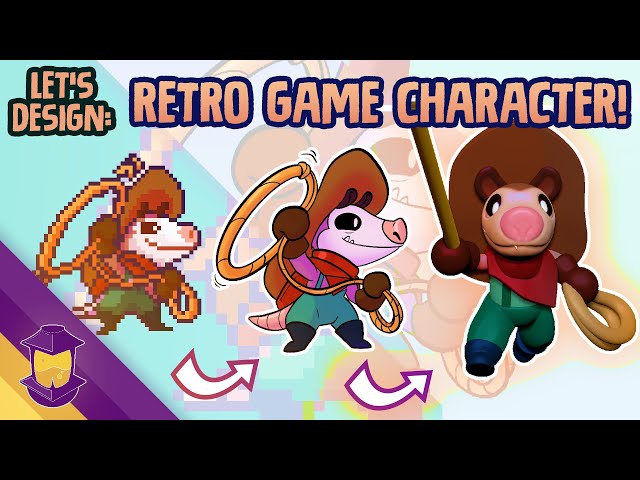The image features the text "Let's Design Retro Game Character" in peach-colored font with a dark navy blue border, accompanied by upward-pointing arrows. Below this, there are three different versions of a character, each displaying an evolution in design style. The character, a possum or wild boar wearing a cowboy hat, green pants, and a brown top coat, appears first in a pixelated retro game style, then in a more detailed and smoother animated version, and finally as a realistic 3D model. Additionally, a purple lamp with yellow light is positioned in the bottom left corner, enhancing the overall retro aesthetic.